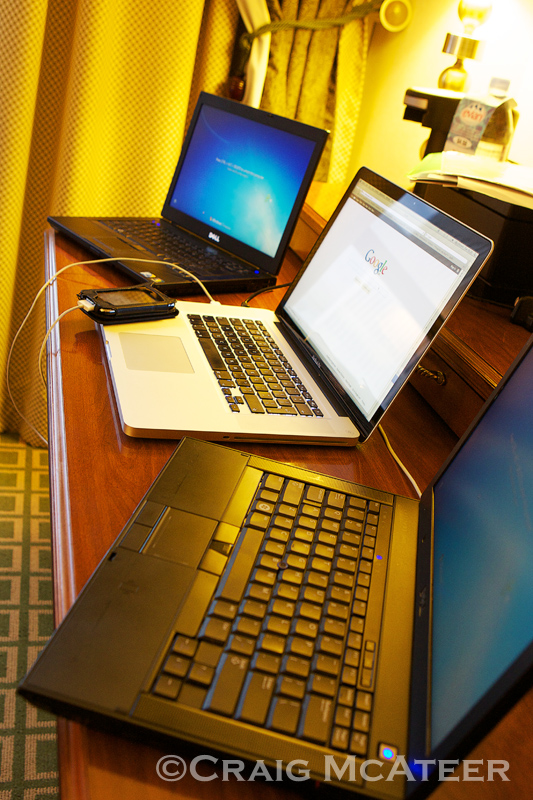In a cozy room illuminated by soft light from the top-right corner, three different style laptops are arranged side-by-side on a brown, possibly mahogany wooden desk. The middle laptop, a silver-gray device with a black top, prominently displays the Google search page. It's connected via a white USB cable to a small cell phone, likely an iPhone, which rests nearby, indicating that it's charging. Flanking this central device are two black laptops, both showing indistinct blue screens that suggest they might be on boot-up or login screens. The desk, slightly cluttered, is backed by yellow curtains and set above a green and yellow patterned floor, adding a touch of domestic ambiance to the scene. Notably, a carpet with green squares and tan outlines softens the area below. The photograph emphasizes the trio of laptops as the main focal point, capturing a snapshot of a workspace perhaps within a hotel room or personal study.